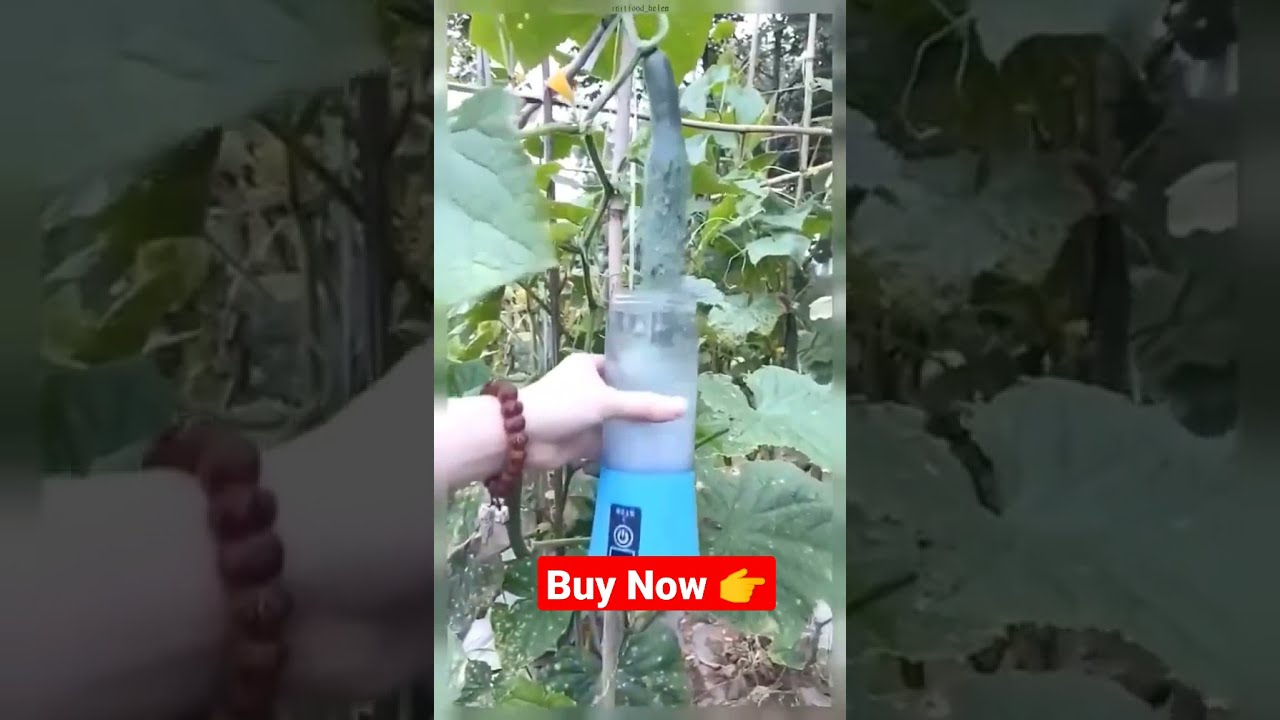The image features a Caucasian person's left hand, adorned with a large brown beaded bracelet, holding a portable blender with a transparent top half containing a grayish liquid and a blue bottom half. This blender has a darker blue sticker with a symbol resembling a power button and a red rectangle with white text that reads "Buy Now," accompanied by a gold hand pointing to the right. The scene is set outdoors, with dense, green foliage and leaves in the background. A green vegetable, possibly a zucchini or cucumber, hangs from a vine and appears to be aimed towards or partially inserted into the blender's opening. The image is divided into thirds: the left showing a close-up of the hand and wrist, and the right showcasing a close-up of the green leaves.